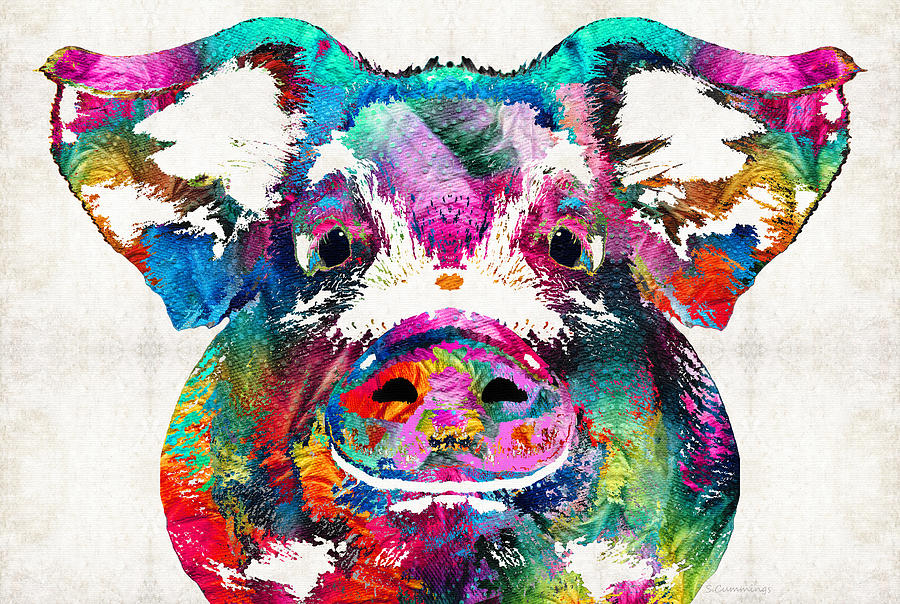This image is a vibrant, psychedelic depiction of a pig's head, facing directly at the viewer. The pig's eyes are two black spots, and its nostrils are small black dots. The multicolored palette includes bright reds, greens, blues, yellows, pinks, purples, oranges, and various shades of white, all blended together in a manner reminiscent of a tie-dye pattern. The background is off-white with varying dimensions of grey, giving it a textured appearance. Notably, white patches embellish areas around the eyes, inside the ears, under the snout, and along the jawline. There are also faint light-colored designs on either side of the pig's head. The image has an overlay or pressed-on style, making it difficult to determine if it's a painting, mural, or digitally created piece.